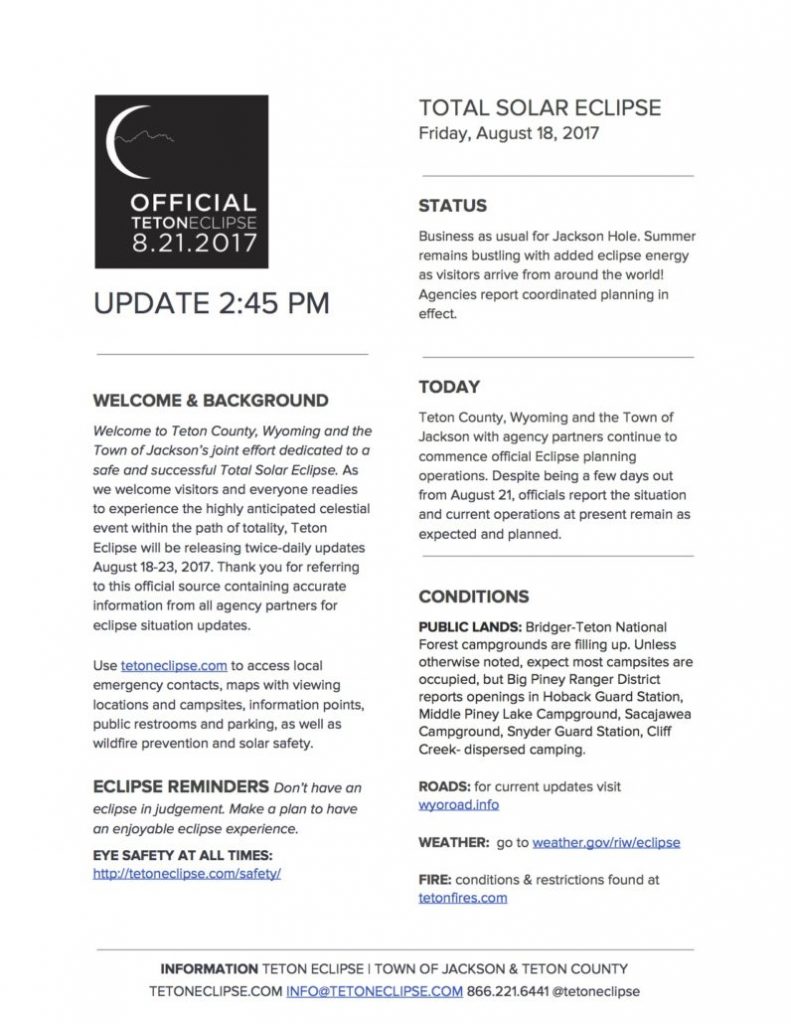The image depicts a section of a website dedicated to the "Official Teton Eclipse," which took place on August 21, 2017. At the top of the website is a small black square featuring a crescent moon in the upper left corner, partially obscured by a line that resembles the upper part of a cloud. Beneath this image, the text reads "OFFICIAL TETON ECLIPSE 8.21.2017."

Directly below the black square, the background turns white, and the text updates the time as "UPDATE 2:45 P.M." in capital letters. Following this, there's a welcome message introducing the joint effort of Teton County, Wyoming, and the town of Jackson, encouraging users to visit "TetonEclipse.com." This hyperlink directs visitors to access important resources such as local emergency contacts, maps of viewing locations, and campsites.

Further down, the website provides safety reminders under the heading "Eclipse Reminders," advising viewers not to "have an eclipse in judgment" and to "make a plan to enjoy an enjoyable eclipse experience." This section is attributed to "Teton Times" and offers a link for more safety information.

On the right side of the webpage, the site lists "Total Solar Eclipse Friday, August 18th, 2017" and provides the current status of conditions related to roads, weather, and fire, with corresponding hyperlinks for each.

At the bottom of the page, the site offers contact details, stating "Information: Teton Eclipse, Town of Jackson and Teton County." The contact information includes the website "TetonEclipse.com," email "info@TetonEclipse.com," and the phone number "866-221-6441."